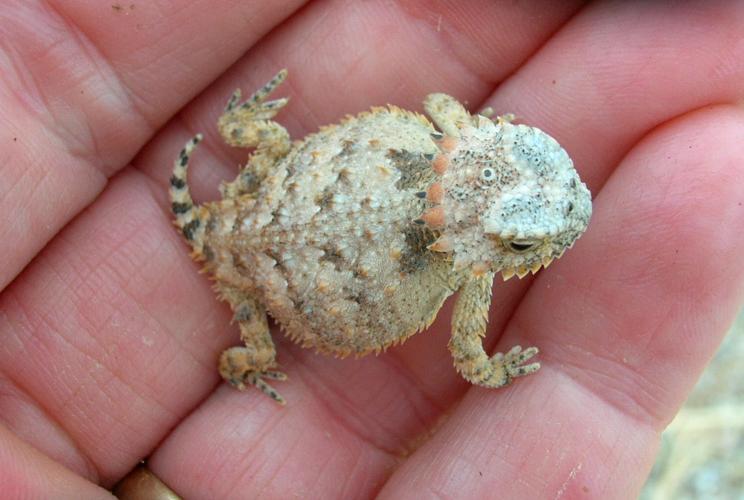In the photograph, a tiny, newborn green horned lizard, also known as a "horny toad," is cradled in the left hand of a white person. The hand is positioned with fingers angled from the bottom left to the top right, with the pinky finger on the right and the pointer finger on the left. The lizard, which is only about the size of two fingers, rests on the second knuckle of the fingers, with its small feet and black-and-yellow tail visible. Its scaly, slightly rounded body features serrated edges lined with tiny, brown horns and white fuzz, indicative of its very young age. The lizard's rugged head is adorned with short, horn-like protrusions, giving it a prehistoric, stone-like appearance, reminiscent of a creature from "The NeverEnding Story." Its unique, almost bead-like texture and the single eye peering up add to its endearing yet curious look.